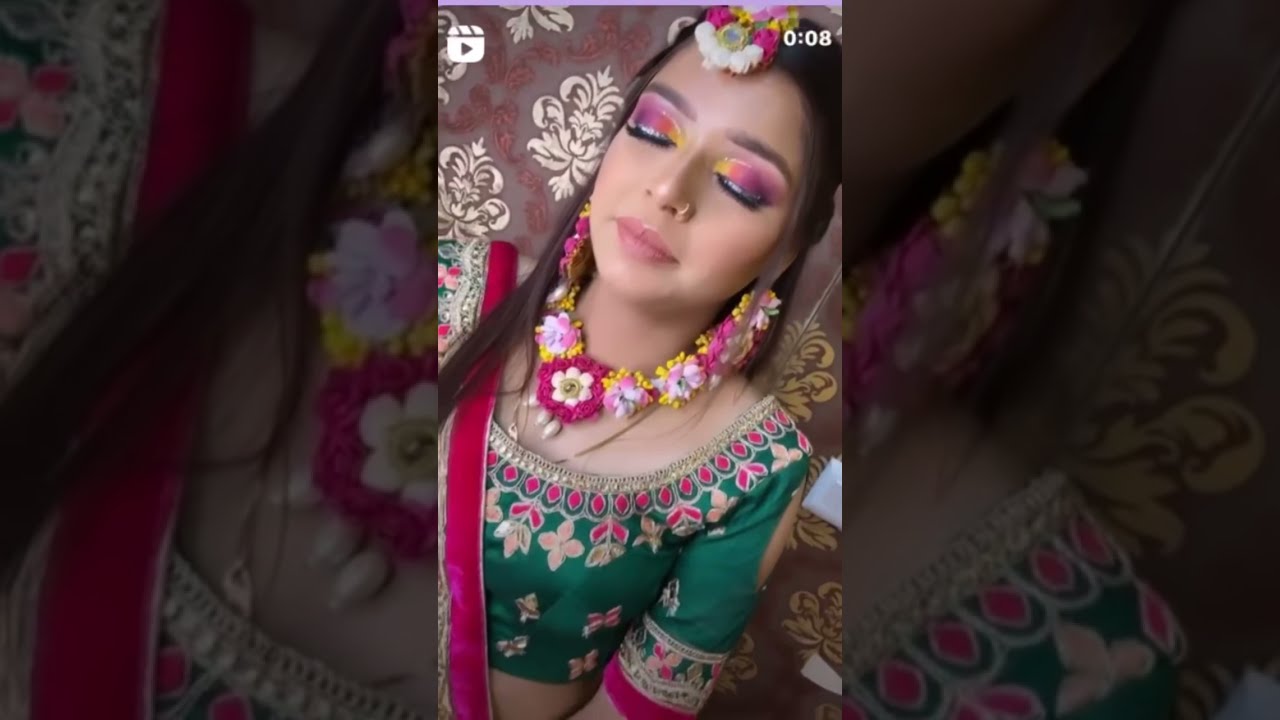In the foreground of the image, a vibrant photograph of a woman dominates the scene, centered precisely in the middle both horizontally and vertically against a slightly blurred background photograph of the same image. The woman appears to be of Middle Eastern or Indian descent and is in her mid-teens to early twenties, exuding a serene and festive aura. She has long, flowing dark hair that cascades past her bodice and some strands lightly fall over her right shoulder. Her eyes are closed, highlighted by bold pink and yellow eyeshadow with white eyeliner, accentuating her eyelids. Her lashes are thick with mascara, and her lips, painted a soft shade of pink, rest gently as if she is in deep meditation or peaceful rest.

Her forehead is adorned with a decorative arrangement of white, yellow, and pink flowers, with similar blossoms forming a necklace around her neck and trailing down from her ears, resembling a lei. Atop her forehead sits a headdress made with pink and white beads complementing the flowers. She sports a gold ring piercing on her nose, adding a touch of traditional elegance. The woman's attire is vibrant and traditional; she wears a green crop top intricately detailed with shades of light and bright pink, trimmed with gold, and decorated with Moroccan-style white patterns. The top has three-quarter sleeves, each hemmed with a decorative pattern of pink and green. Draped over her shoulder is a pink sash, adding to her culturally rich ensemble and emphasizing her bare midriff.

The colorful background behind her, composed of pink, white, and gold hues, appears to be part of a Middle Eastern rug or cushion, further accentuating the ethnic and festive quality of the scene. This exceptional photograph captures not only the beauty and essence of cultural attire but also a moment of serene introspection, as reflected by the woman's peaceful expression and closed eyes.